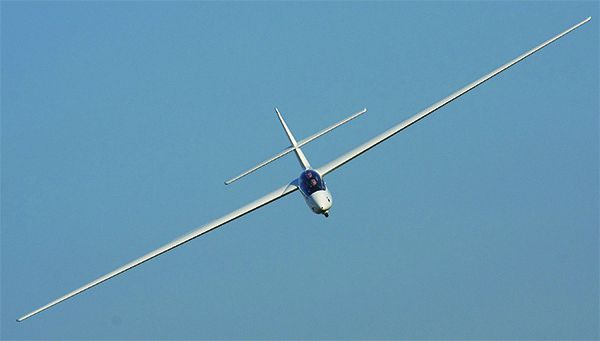The image features a small, white or light silver plane gliding diagonally across a clear, blue sky. Its long, thin wings stretch from the bottom left corner to the top right corner of the frame, showcasing a remarkable span for such a compact aircraft. The narrow fuselage houses a small cockpit with what appears to be space for two passengers, one seated in front of the other, visible through a large, clear window. The tail of the plane extends outward, finishing in a smaller, perpendicular tail wing that resembles a cross. The composition is stark and minimalistic, placing emphasis solely on the elegant aircraft and its distinctive long wings against the crisp, cloudless background.